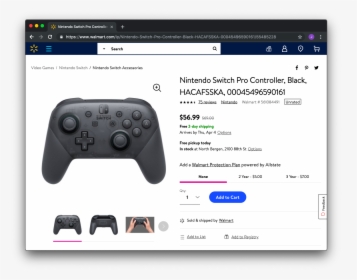This is a detailed screenshot from Walmart's online store. Located at the top left corner, the Walmart logo, featuring a yellow flower petal symbol, is prominently displayed. The focal point of the image is the Nintendo Switch Pro Controller in black, priced at $56.99. The controller's primary image is centered and slightly to the left, with the product name and price listed to its right. Beneath the main image are three smaller thumbnails showcasing different views of the controller: a back view, a front view, and one with hands holding it. The browser displaying the webpage is in dark mode, evident by the black color of the top bar, which also shows that only one tab is open. Lastly, a blue "Add to Cart" button is visible, along with an option to select the quantity, which is currently set to 1.